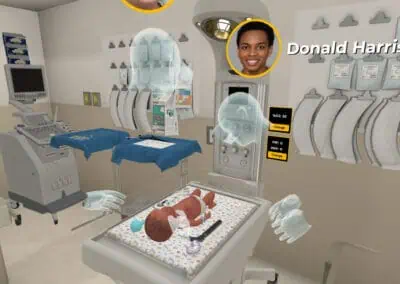This rectangular image, approximately two inches wide and one and a half inches high, appears to be a detailed still from a virtual reality simulation set inside a hospital room. The focus of the image is a low-lying exam table positioned centrally at the bottom, on which lies a baby of Caucasian descent, dressed in a white diaper and resting on a white pad adorned with animal images. Surrounding the baby are transparent whitish-gray heads and hands, representing medical personnel with no attached bodies, peering down at the infant. 

In the room's background, the walls are a mix of white and cream colors, and to the left, there's an array of medical equipment including a large computer on wheels with a big monitor. Additional medical bags and clipboard-like items hang from a gray wall. 

Above the baby, toward the top and slightly to the right, is a yellow-outlined circle containing the photograph of an African descent individual, accompanied by the name "Donald Harris" in white print. This suggests that Donald Harris may be one of the participants or operators in this virtual reality simulation, likely used for practicing medical procedures.

The overall scene resembles a high-tech, graphically represented surgery or medical training game, emphasizing the interactive and educational aspects of the simulated environment.